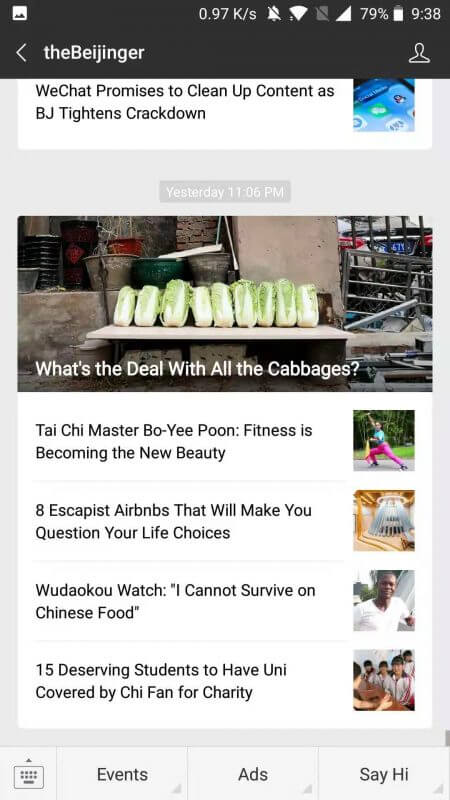A detailed caption for the image could be:

"A comprehensive view of a smartphone screen displaying 'The Beijinger' app. At the top, familiar smartphone icons including a notification bell, battery percentage, and the current time are visible. Below these, the app interface begins with a prominent heading 'The Beijinger' and an outline icon for accessing user profiles. The screen showcases a series of news headlines and articles. The first headline reads, 'WeChat promises to clean up content as BJ Titans crackdown,' timestamped at 'yesterday, 11:06 PM.' This is followed by an intriguing headline, 'What's the deal with all the cabbages?', accompanied by an image of numerous cabbages closely arranged on what appears to be a street-side table or a spot behind a restaurant.

Further down, another article titled 'Tai Chi master Bo Yipun: fitness is becoming the new beauty,' features an image of a person exercising. The subsequent headline, 'Eight escapist Airbnbs that will make you question your life choices,' includes a photograph of a well-furnished room, promising a tempting retreat. 'Wudacca Watch: I cannot survive on Chinese food,' shares a man's story with an image of him in a white t-shirt. Lastly, '15 deserving students to have uni covered by Chai Fan for charity,' highlights a noble cause with an image of school students.

At the bottom of the screen, navigation tabs labeled 'Events,' 'Ads,' and an option 'Say Hi' offer additional functionalities. The interface features a light-colored background with contrasting black text, ensuring readability and user-friendly navigation throughout the app."